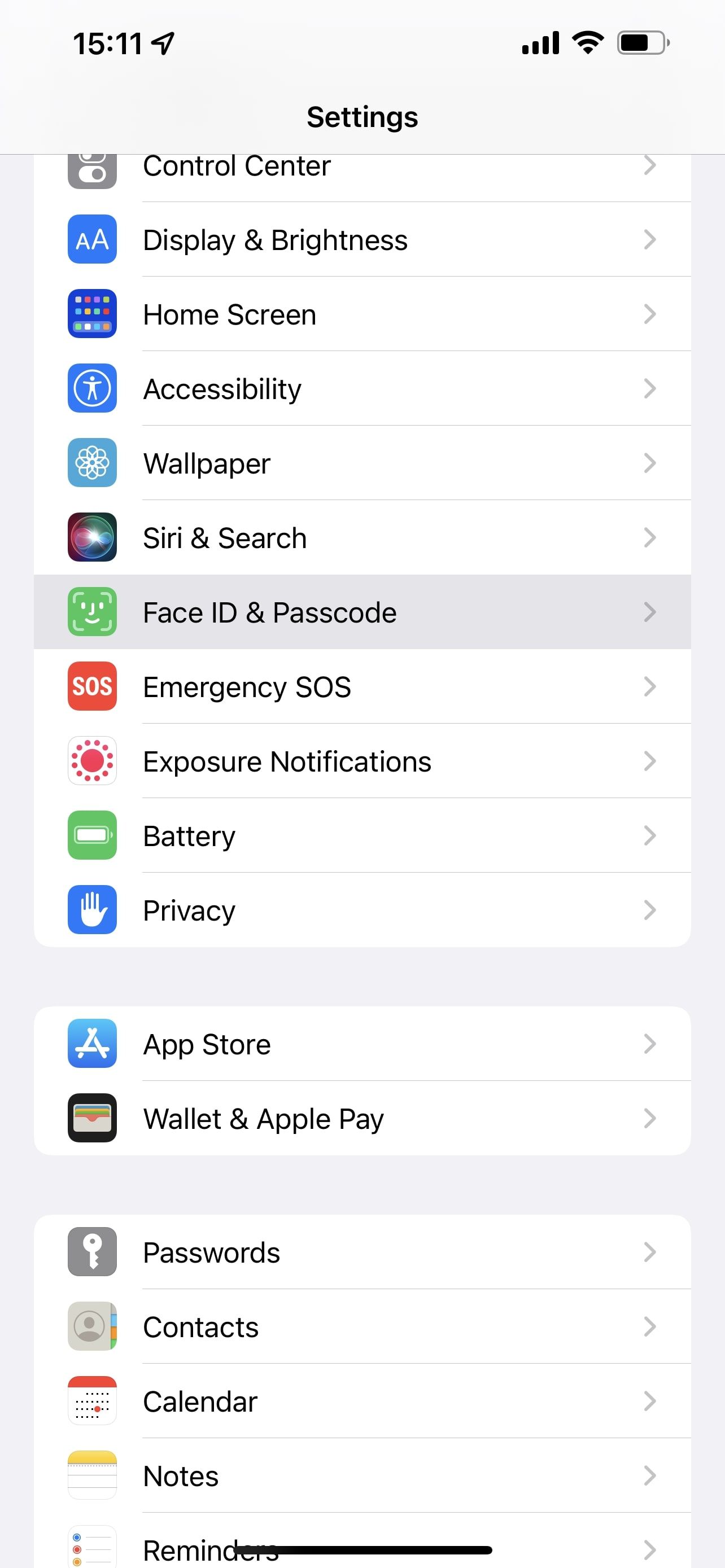This portrait-oriented screenshot displays a detailed view of an iPhone settings menu, segmented into numerous rows and sections. At the very top of the screen, a light gray stripe extends from the upper left-hand corner to the upper right-hand corner. The upper left-hand corner displays the time "15:11," while the upper right-hand corner shows a battery icon with slightly more than 50% charge remaining. 

Directly beneath this stripe, the next row features the word "Settings" in bold, centered black font. Below it, the partially scrolled-up menu lists "Control Center." As the user scrolls through the settings, each row displays a corresponding icon on the left. 

The next rows include: “Display & Brightness,” “Home Screen,” "Accessibility," "Wallpaper," "Siri & Search," and currently highlighted in gray, "Face ID & Passcode." Clicking the right arrow at the end of this row would navigate to the "Face ID & Passcode" page.

Following these rows, you will see "Emergency SOS," "Exposure Notifications," "Battery," and "Privacy." Another light gray stripe introduces a new set of rows, including "App Store" and "Wallet & Apple Pay." Again separated by a gray stripe, the subsequent rows list “Passwords,” “Contacts,” “Calendar,” “Notes,” and “Reminders.” Each setting is distinctly separated by thin gray lines for clarity.